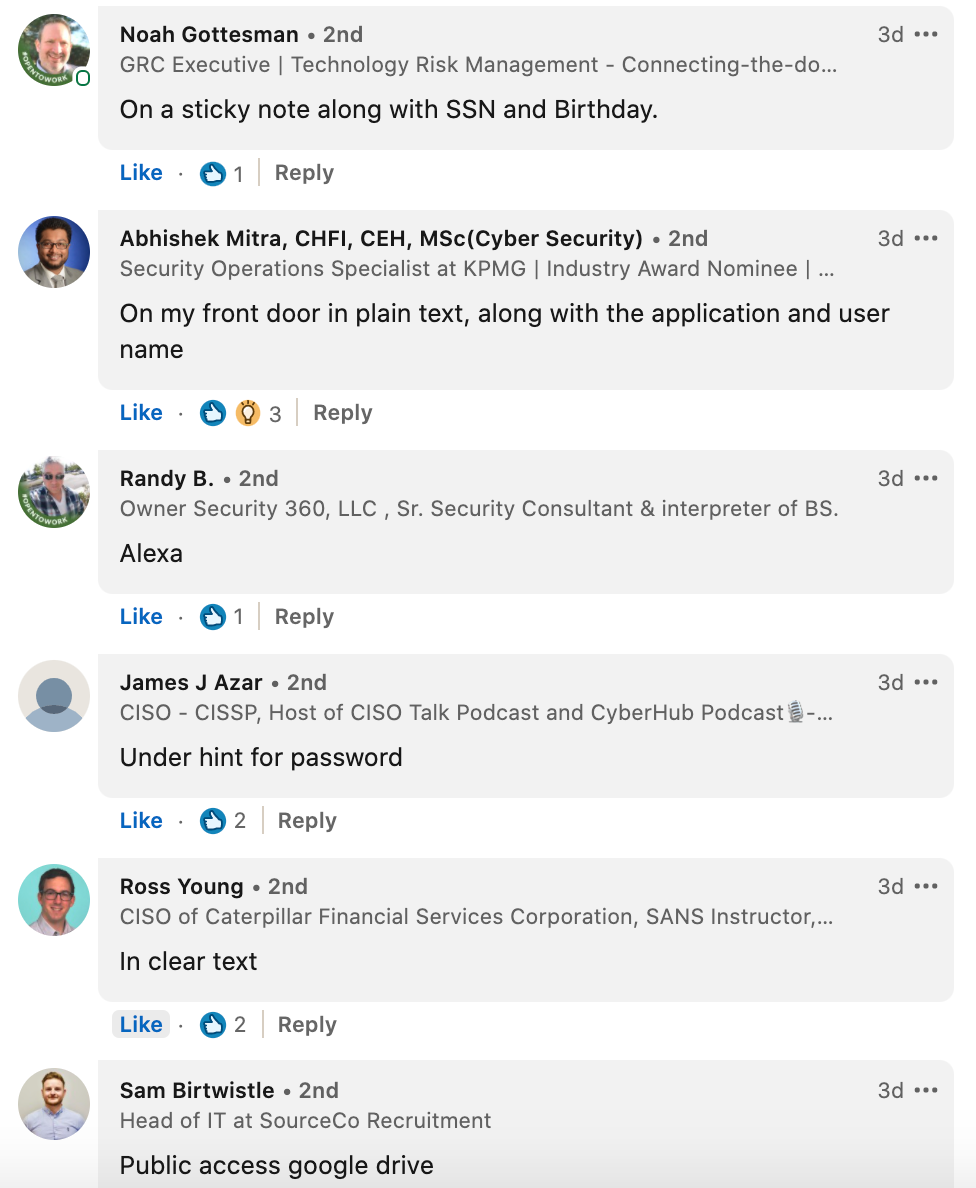The image is a detailed screenshot of a virtual meeting or webinar interface, featuring multiple participants each displayed in individual boxes. Starting at the top left, the first box is labeled with the name "Noah Gotsman." Each participant’s box includes a circular profile picture. Noah Gotsman's profile picture depicts a white man staring at the camera under bright, sunny conditions. 

To the right of Noah's box, the next participant's name and details are somewhat obscured but mentioned as "second to the right of his name." Below this, the text reads "GRC executive technology risk management connecting the do," followed by a sticky note annotation with "SSN and birthday."

In the second row, the box to the left features "Abhishek Mitra." His comment, written in plain text, mentions something about "on my front door," along with "application and username."

In the center of the image, the third box showcases "Randy B." His comment is simply "Alexa."

The fourth box features "James J. Azar," whose comment reads "hint for password."

Towards the bottom, the fifth box displays "Ross Young," with his comment stating "in clear text."

At the very bottom, the last box displays the name "Sam Burt Whistle" and his comment, "public access Google Drive."